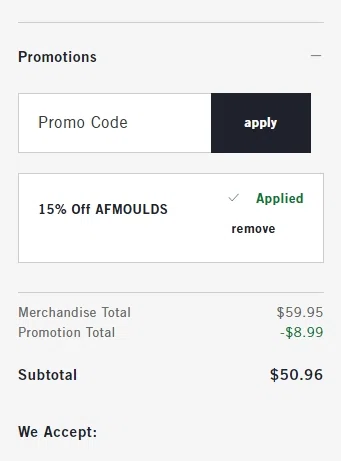The image features a light blue background with a design intended for an online shopping checkout interface. At the top, a thin blue line displays the word "Promotions." Below it, a small white box labeled "Promo Code" includes a black button that says "Apply." Another white box underneath shows a promotional code "15% off AFMOLDS," accompanied by a green checkmark next to the word "Applied" in green text alongside a black "Remove" option.

Further down, another thin line separates the promo section from the order summary. The merchandise total is listed as $59.95. A promotional discount subtracts $8.99 from the total, resulting in a subtotal of $50.96. At the bottom, a text indicates that the system accepts various payment methods. This detailed breakdown highlights the successful application of the "15% off AFMOLDS" promotion.